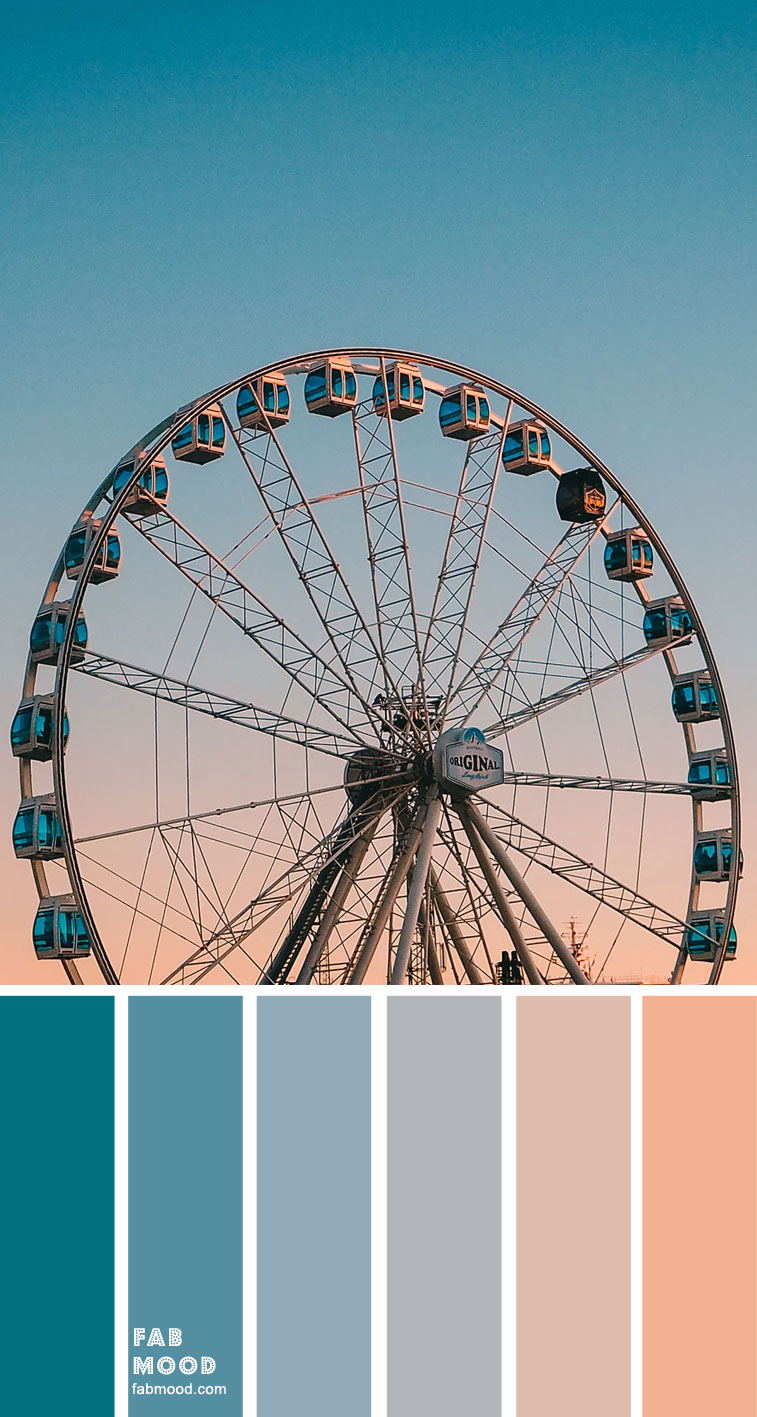The image features a prominent, tall rectangular photograph of a large Ferris wheel, possibly the London Eye or Seattle Wheel, made of silver metal with silver cars that have blue-tinted windows and doors. The Ferris wheel, located at the top of the image, is slightly off-center to the left and almost touches the edges of the photograph. The sky transitions from a bright blue at the top to a soft orange hue at the bottom, creating a stunning gradient reminiscent of a sunset. In the middle of the Ferris wheel, there is a blue and white sign with a logo on it. Below this photograph, separated by thin white borders, are six solid color rectangles that match the gradient hues of the sky above. These rectangles, resembling paint swatches, range from a deep teal on the left to a peach color on the right, and the second rectangle from the left is marked with the white text "Fab Mood, fabmood.com."